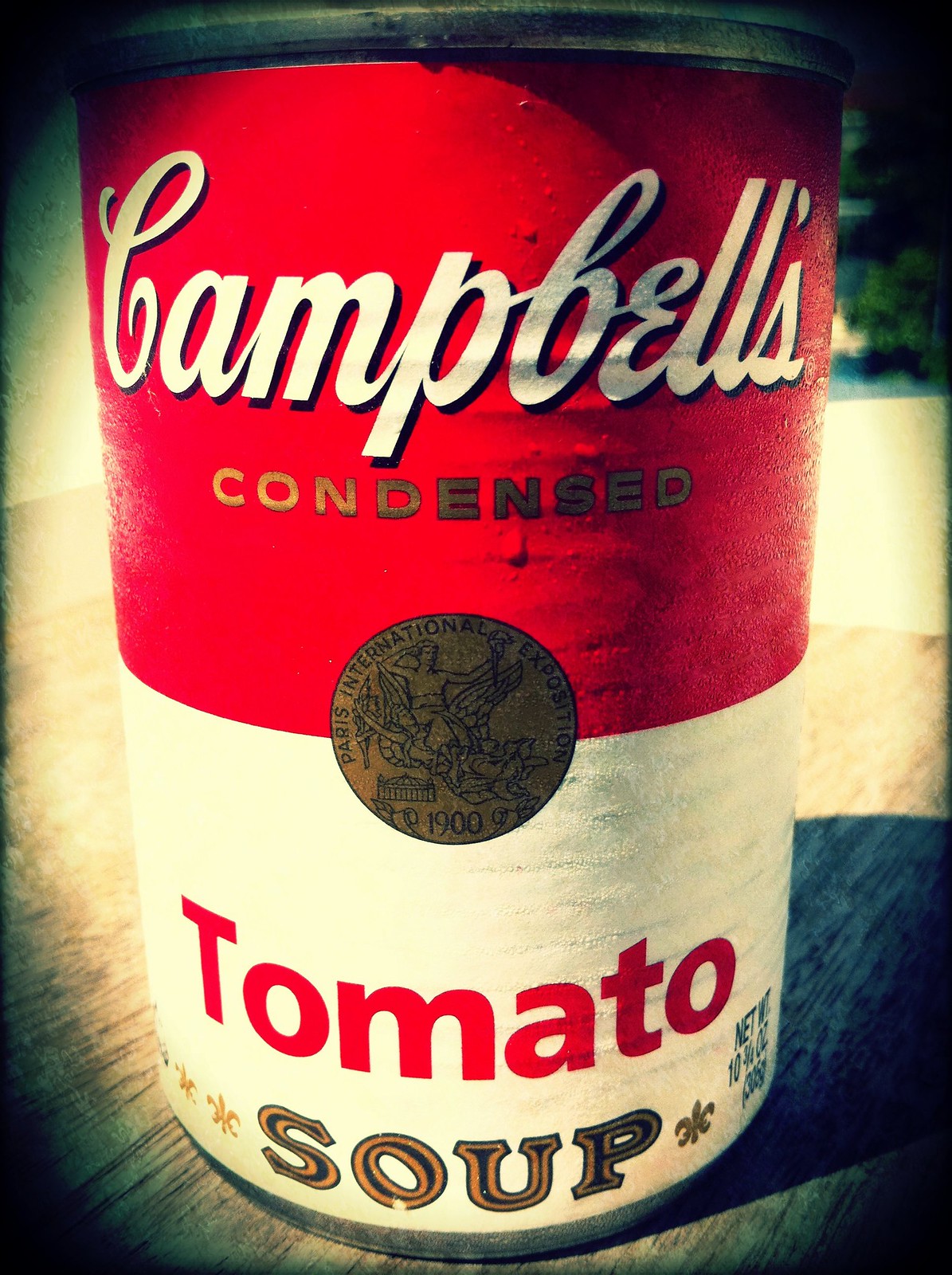A nostalgic photograph capturing a classic can of Campbell's Condensed Tomato Soup, a timeless staple in many households for over a century. This iconic red and white can of soup is adorned with an intricate gold medallion, lending it a vintage charm. The branding is distinctly recognizable: the script of "Campbell's" gleams in white, while "Condensed" is set in a sophisticated gold. The word "Tomato" stands out in a vibrant red font, and "Soup" is elegantly framed in gold and black. This image conjures fond memories of family meals, particularly the beloved pairing of tomato soup and grilled cheese sandwiches.